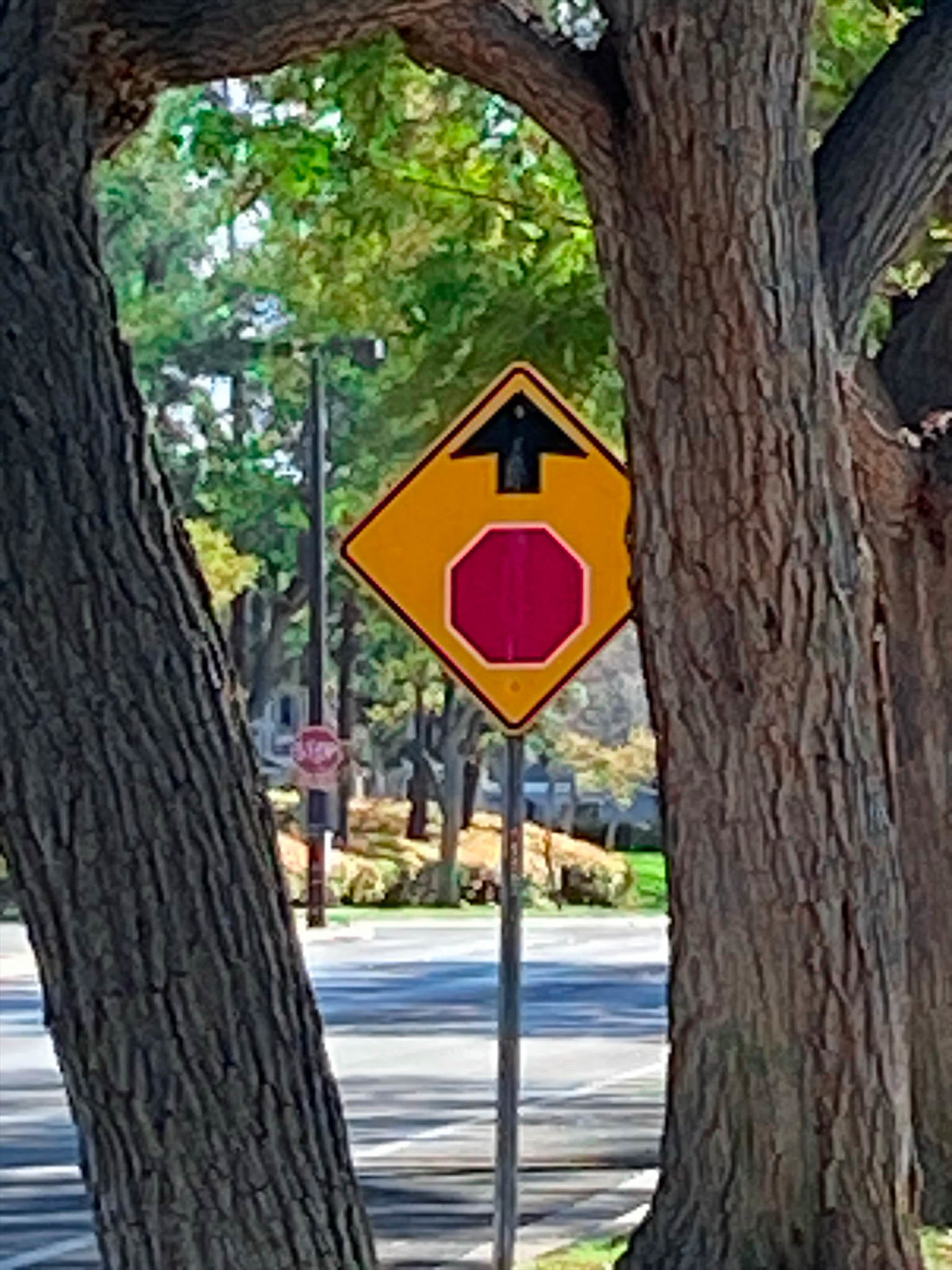The photograph captures a street scene centered around a diamond-shaped road sign mounted on a gray pole, positioned between two trees. The tree on the left leans slightly, with dark gray bark, while the tree on the right stands upright with a light brown trunk. Both trees are only visible from their bases and stretch vertically out of the frame. The road sign features a red hexagon with a white border and a black arrow pointing upwards. Above this sign, green leaves partially obscure the sky. Below and extending into the distance, the gray road leads to a stop sign and a few houses further along. The image blends natural and urban elements, portraying an everyday street scene with nuanced details.